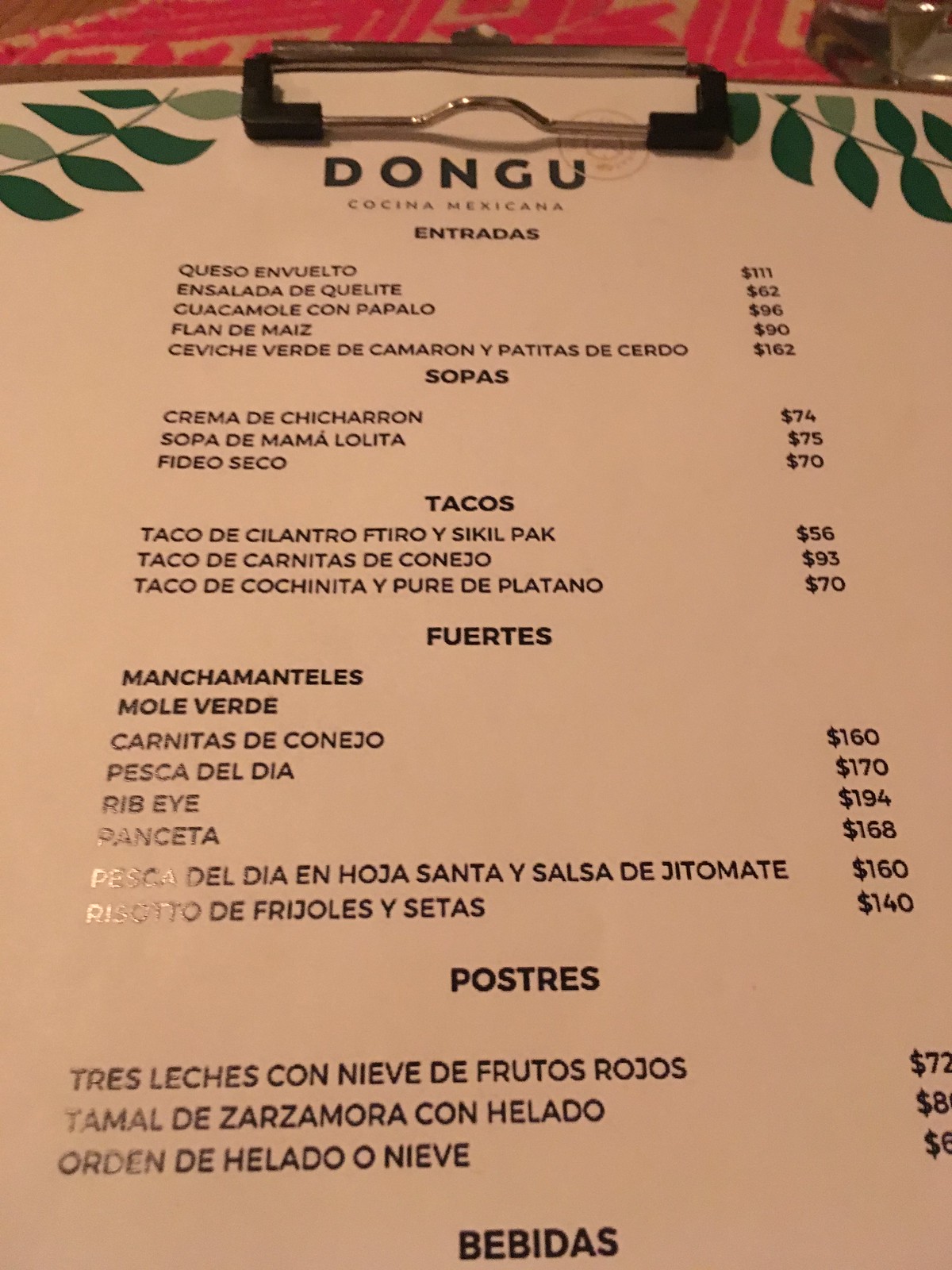In this first-person perspective image, a laminated A4 menu is held to a wooden surface using a steel clasp positioned in the center. The menu is predominantly white and is adorned with delicate vine and leaf illustrations in the top corners. The wooden surface is minimally visible, with just a tiny sliver exposed at the top left corner. Below the menu, a faint pink and white patterned tablecloth is partially observable, indicating that the setting is likely a restaurant. The tablecloth covers around one-tenth of the image and is somewhat difficult to discern. Meanwhile, the table itself appears to be wooden. A hint of a plant decoration is noticeable in the top right corner, suggesting a leafy element adds to the restaurant's ambiance.

Printed prominently in bold black text at the center of the menu are the words "Dongu Coquina Mexicana". The menu headers are in Spanish, organized as follows: "Entradas" (Entrees), "Sopas" (Soups), and "Tacos". Additional sections include "Fuertes" (Main Courses) and "Bebidas" (Drinks). The majority of the menu remains out of frame, but the prices listed in the right-most column are visible, with specific amounts in Mexican pesos: $111, $62, $96, $90, $162, $74, $75, $70, $56, $93, $70, $160, $170, $194, $168, $160, and $140. The "Postres" (Desserts) section is also listed but the pricing for these items is not captured in the image. This menu provides insight into the restaurant's offerings and pricing structure.